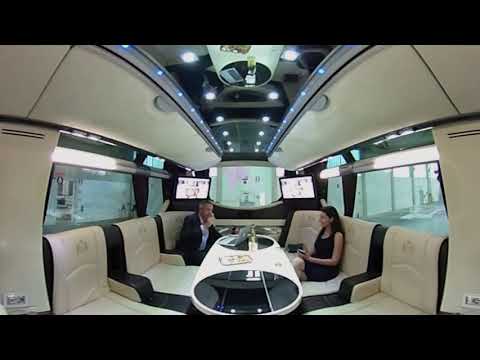The image showcases the interior of a luxurious travel vehicle, possibly a high-end van, limousine, or elegant train car. The space, despite being compact, exudes opulence and functionality, resembling a modern conference room. At the center of the room, an oval-shaped table, in a striking black and white design, is surrounded by six plush leather chairs—three on each side. Two of these chairs are occupied by a man in a suit and a woman in a black dress. Both individuals are dressed in business casual attire, suggesting a professional setting. Behind the chairs, large windows line the walls, offering glimpses of the exterior. The ceiling is adorned with recessed LED lights, creating a sophisticated ambiance, while the back wall features two televisions—one mounted on each side. Adding to the room's modernity, a laptop and a bottle are placed on the table. The overall setting embodies a blend of luxury and practicality, ideal for business meetings on the go.